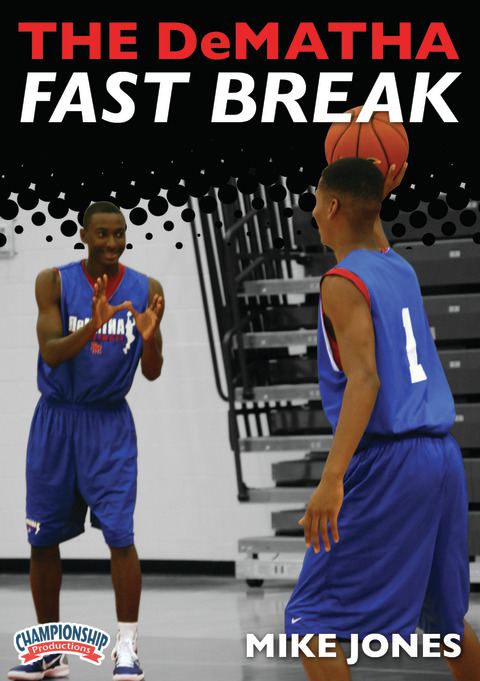This advertisement poster for a basketball event features a dynamic photograph of two men in bright blue Nike basketball uniforms with red accents around the neck and sleeveless sleeves. The rectangular poster, which is taller than it is wide, shows the man on the left facing the camera with a smile, arms raised as if ready to catch a ball. His uniform has some writing on the front, partially obscured by his raised hands. The man on the right is seen from the back, holding a basketball high in his right hand, with the number one visible on his jersey. They appear to be on a court, with a possible rack of equipment or chairs in the background. The top of the poster features the text "V. DeMatha" in red and "Fast Break" in white against a black background. At the bottom left, a white banner with blue lettering says "Championship Productions," and a red banner with white lettering next to it reads "Productions." On the bottom right, the name "Mike Jones" is prominently displayed in white.